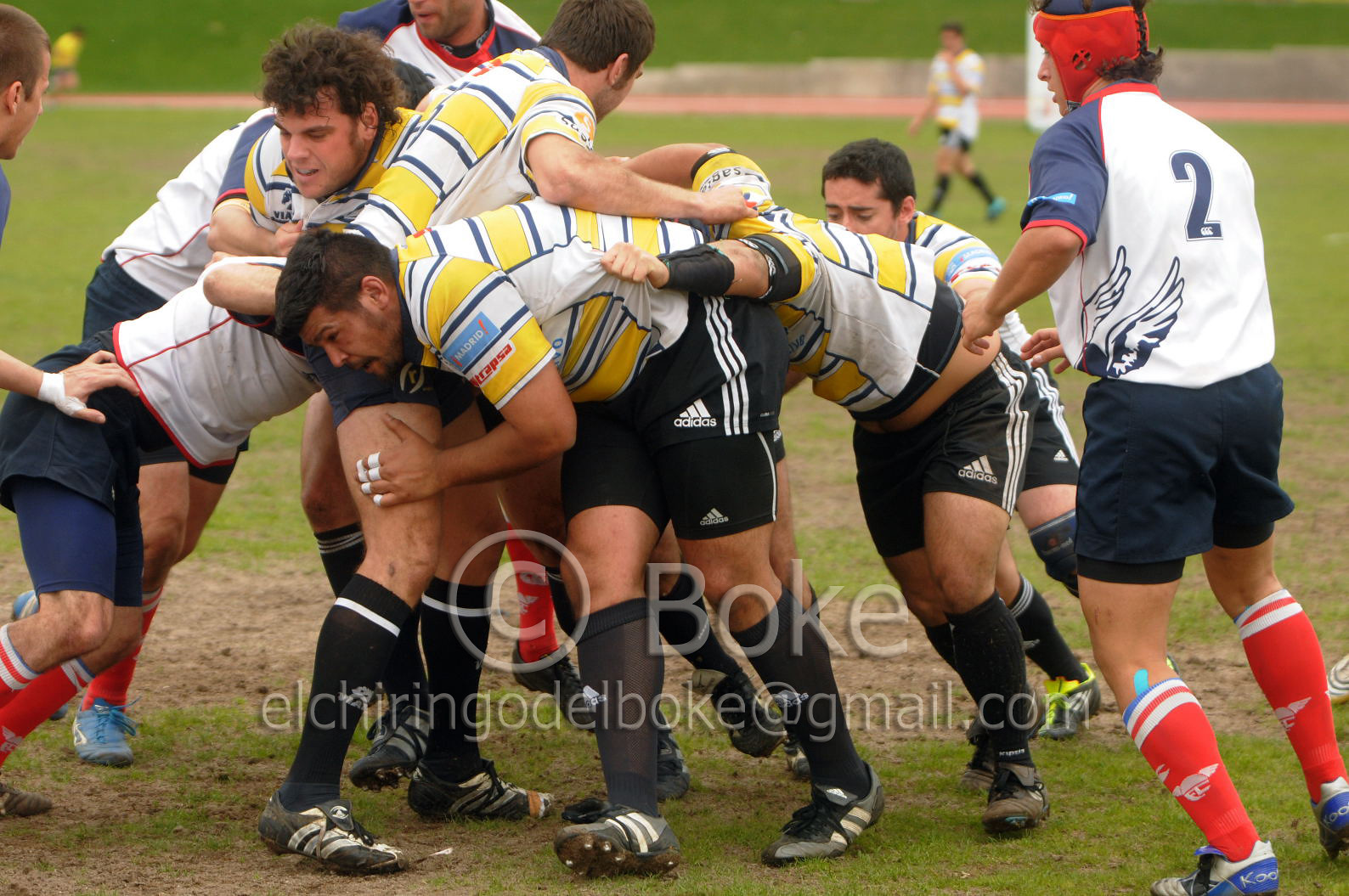This photograph captures an intense moment during a rugby match, prominently featuring a sizable watermark attributed to the author, with the copyright marked as "Boke" (B-O-K-E) and the email address elchirin.godelboke@gmail.com. In this dynamic scene, approximately ten players are vigorously contesting for possession of the rugby ball. One team is clad in yellow and white striped jerseys, while the opposing team sports navy blue and white jerseys. The background reveals additional players, all situated on a muddy, rain-soaked grass field, indicative of the recent weather conditions and the physicality of the game. The players' expressions are intensely focused, conveying the high stakes and competitive nature of the match.